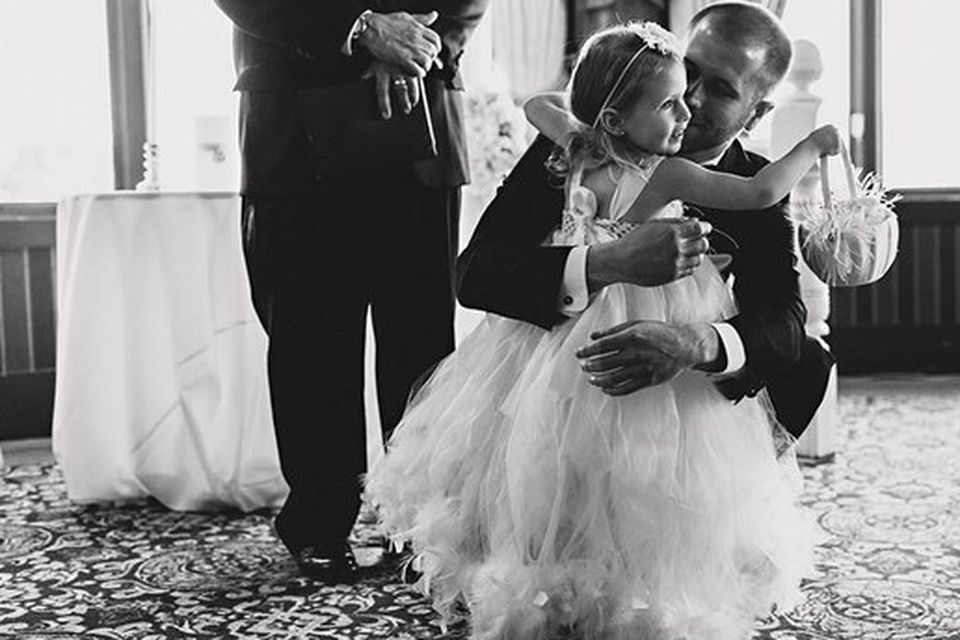In this black-and-white photograph, a man in his 30s, dressed in a formal tuxedo, crouches down to affectionately embrace and kiss a young girl, likely around six or seven years old. The girl, possibly a flower girl given her role, is clad in a fluffy, lacy white dress and adorned with a bonnet-like headpiece. She holds a small basket, possibly used for wedding items, that contains thin pieces of straw or feathers. Behind them stands another man, partially visible from the torso down, with his hands clasped in front of him, dressed in a formal suit. Further back, a table draped with a white tablecloth and adorned with ornaments, likely for a wedding cake or gifts, is positioned near wood-paneled half-walls and windows. The oriental-style carpet on the floor adds to the elegant setting, reinforcing the wedding atmosphere depicted in this monochromatic image.